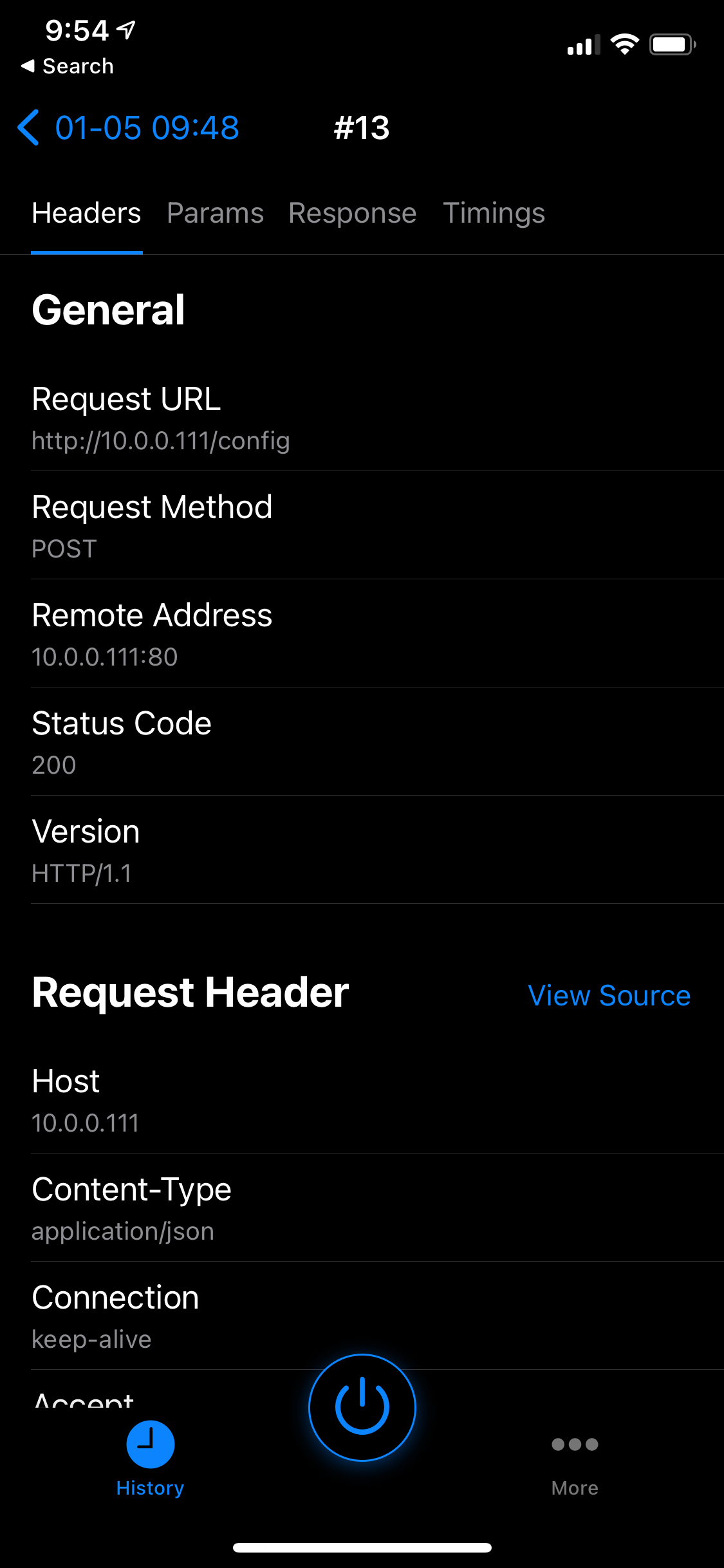The image is a screenshot of a phone settings interface, displaying specific technical details. The background of the screenshot is black. At the top of the screen, the time is displayed as "9:54," accompanied by an arrow icon, a moderate signal indicator, a high Wi-Fi signal icon, and a battery icon showing approximately 100% charge.

Beneath the top bar, there is a search option. Following this is the date and time displayed as "January 5th, 9:48," written in blue letters, with the number "13" adjacent to it. Below this, there is a menu with four items: "Header," "Params," "Response," and "Timings."

In bold white letters, the word "General" is written, indicating the general settings section. The general settings include several options listed as "Request URL," "Request Method," "Remote Address," "Status Code," and "Version."

Further down is another header labeled "Request Header," and to its right is an option labeled "Use Source." Under the "Request Header" section, there are four items, although only three are fully visible: "Host," "Content Type," "Connection," and partially visible "Accept," where some letters are cut off at the bottom.

At the bottom of the screen, there is a menu button displaying three options: a link to the history on the left, a central button for file toggling, indicated as "File On/Off," and a "More" option on the right.